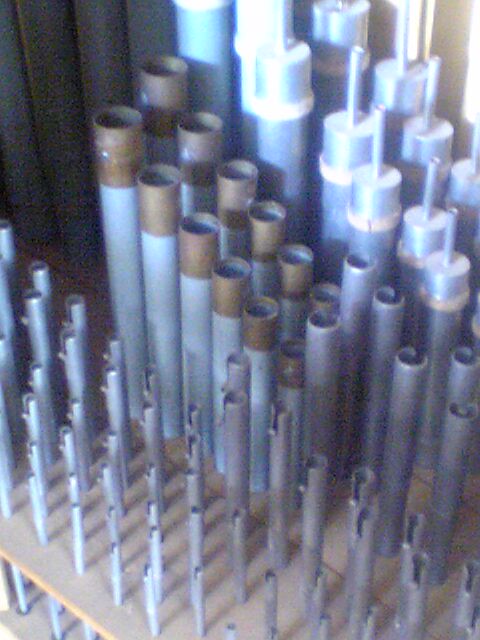This image showcases a meticulously arranged collection of metal and cardboard cylinders of varying heights and diameters, standing vertically on a wide, natural-colored wooden board with numerous holes, functioning almost like a pegboard. In this arrangement, some of the metal cylinders have distinct features such as brown or gold tops, and some possess small steel ledges as if designed to hold or separate items. The skinnier, silver rods are in the foreground, some adorned with stacked circular silver elements. Taller, thicker cylinders, including one with a gold-tipped section, dominate the background. A uniquely shaped tube with a skinny extension is also visible among the larger rods. The overall scene appears organized and intentional, with the wooden panel's holes providing a versatile framework for this diverse assembly of cylinders.